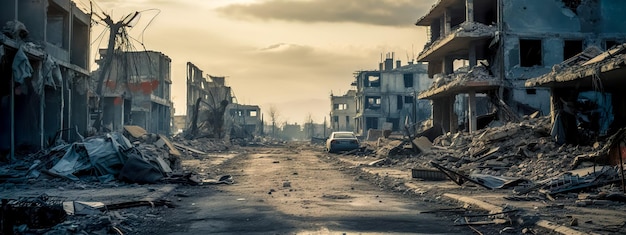The image depicts an outdoor scene of a city in utter destruction, likely caused by a severe storm or bombing. The devastation is widespread, with buildings on both sides of a central street torn apart and reduced to rubble. The structures are stripped of their roofs and interior walls, leaving only skeletal frameworks and crumbling facades. Debris litters the street, which runs from the foreground to the middle of the image. On the left, a three-story building shows exposed floors with completely shattered windows and walls. The right side mirrors this destruction with more buildings reduced to piles of rubble. A single abandoned car is parked on the right side of the street, its orientation facing away from us. The scene is enveloped in a gray and beige haze, with an ashy, smoky atmosphere that adds to the overall sense of desolation and chaos. The sky above is filled with dark, ominous clouds, contributing to the eerie and apocalyptic feel of the scene.